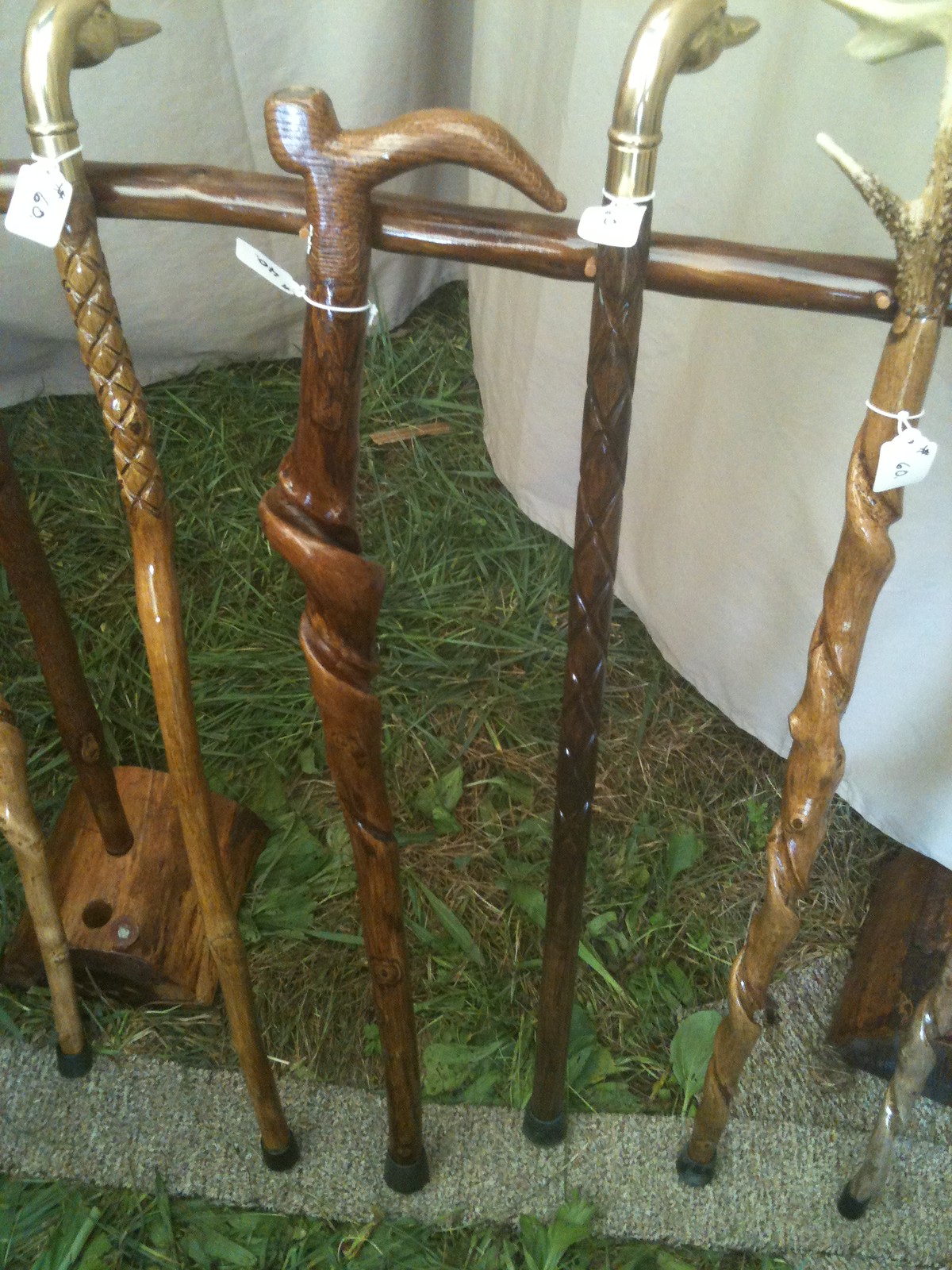This portrait-oriented color photograph, taken outdoors, depicts an array of intricately designed walking sticks on display, likely for sale at an outdoor market or stall. The walking sticks, polished to a shiny finish that highlights the grain of the wood, are varied in style. Some feature elegant, twisted designs, while others are adorned with ornate handles, including metallic duck heads and carved wooden tops. They are leaning against a horizontal wooden branch, with their black rubber feet resting on the trampled green grass. Each walking stick is marked with a small white tag tied around the top, some clearly showing the number "60," indicating their price. In the background, off-white fabric, possibly from a tent or canopy, adds to the open-air market ambiance. Although the photograph predominantly focuses on four walking sticks, additional canes are partially visible, hinting at a wider selection.